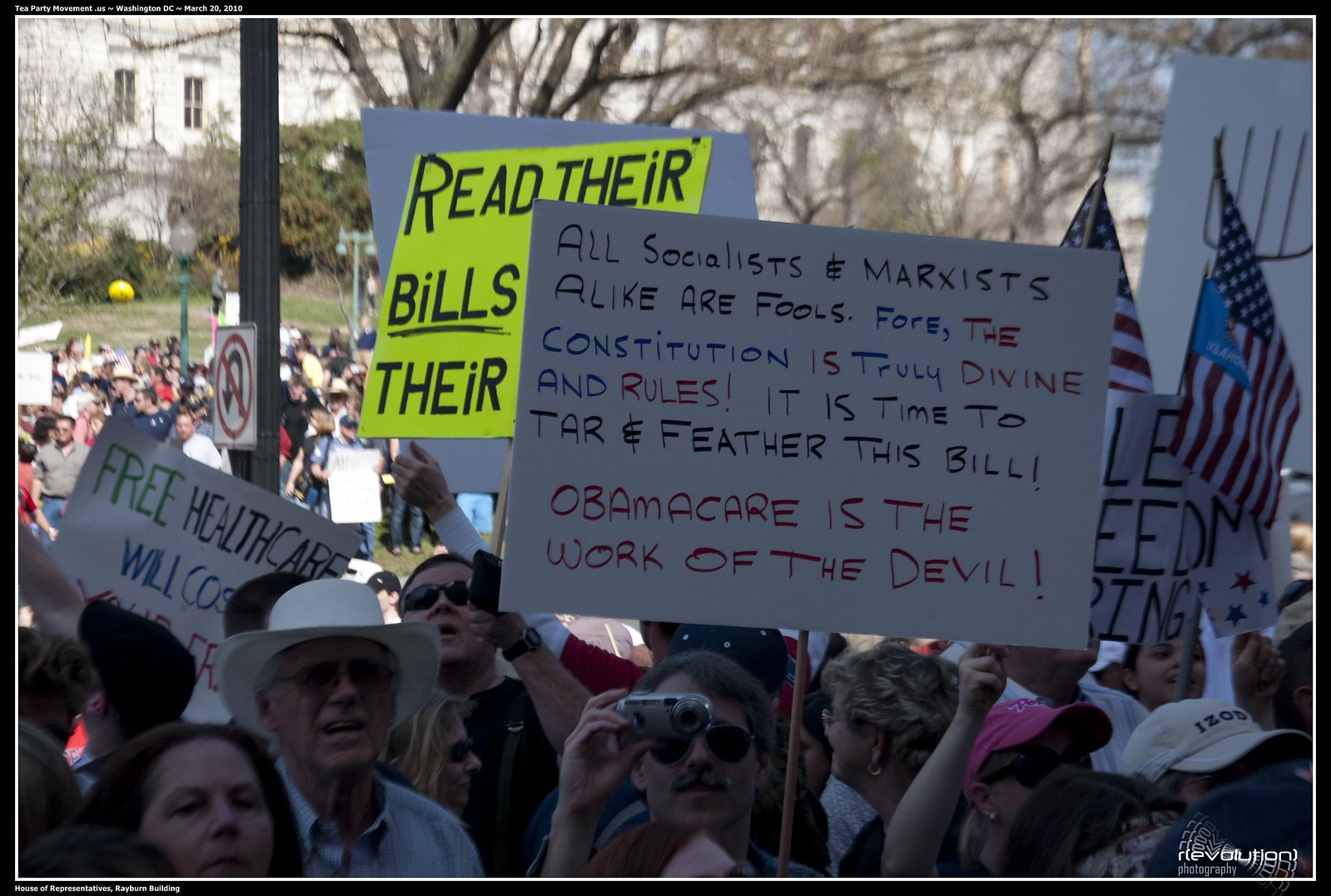The photograph captures a large protest, likely taking place outside a prominent white government building, possibly in Washington D.C. The image is somewhat out of focus and shadowy, primarily showing a crowd of older, predominantly Caucasian individuals. Among the handmade, brightly colored poster board signs being held up, several are clearly readable. One prominent sign reads, "All socialists and Marxists alike are fools, for the Constitution is truly divine and rules! It is time to tar and feather this bill! Obamacare is the work of the devil." Other signs reference healthcare, socialism, and issues with Obamacare. The crowd is dense, with various flags visible, set against a backdrop of trees and a No U-Turn road sign.